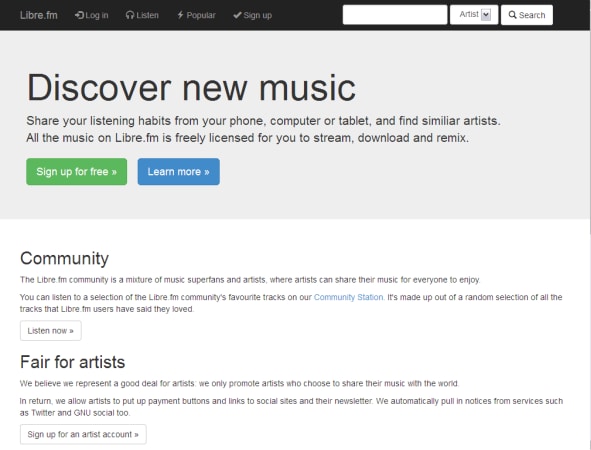This image is a screenshot of the Libre.fm platform, showcasing a structured and detailed interface. 

At the top of the image, there's a prominent black bar featuring the main navigation menu. Starting from the left, the menu begins with the Libre.fm logo rendered in a subtle gray text that nearly blends with the black background. Adjacent to the logo are several navigation options: a login icon, a “Listen” link, a “Popular” link adorned with a lightning bolt icon, and a “Sign Up” option accompanied by a checkmark icon. 

To the right of these options is a search area that includes a blank search field with a dropdown menu labeled "Artists." This search function is complemented by a search button that features a magnifying glass icon on a light gray background.

Beneath this black navigation bar is a light gray hero section. Dominating this section is a bold headline that reads "Discover New Music," which is the largest text in the image. Below this headline is a subheading formulated in a slightly smaller font: “Share your listening habits from your phone, computer or tablet, and find similar artists. All the music on Libre.fm is freely licensed for you to stream, download, and remix.” 

Further down within the hero section are two prominent call-to-action buttons. On the left, the green “Sign Up for Free” button with rounded corners invites new users to join. Next to it is a blue “Learn More” button, also with rounded corners, for those seeking additional information.

The section transitions into a white background, dividing the content into two distinct rows. The first row is labeled “Community,” containing three lines of explanatory text followed by a “Listen Now” button. Below it is the “Fair for Artists” section, also with three lines of descriptive text, and a “Sign Up for Artist Account” button designated for artists.

This detailed structure provides a comprehensive overview of the Libre.fm platform's interface, emphasizing user navigation, discovery, and engagement with both music and community features.